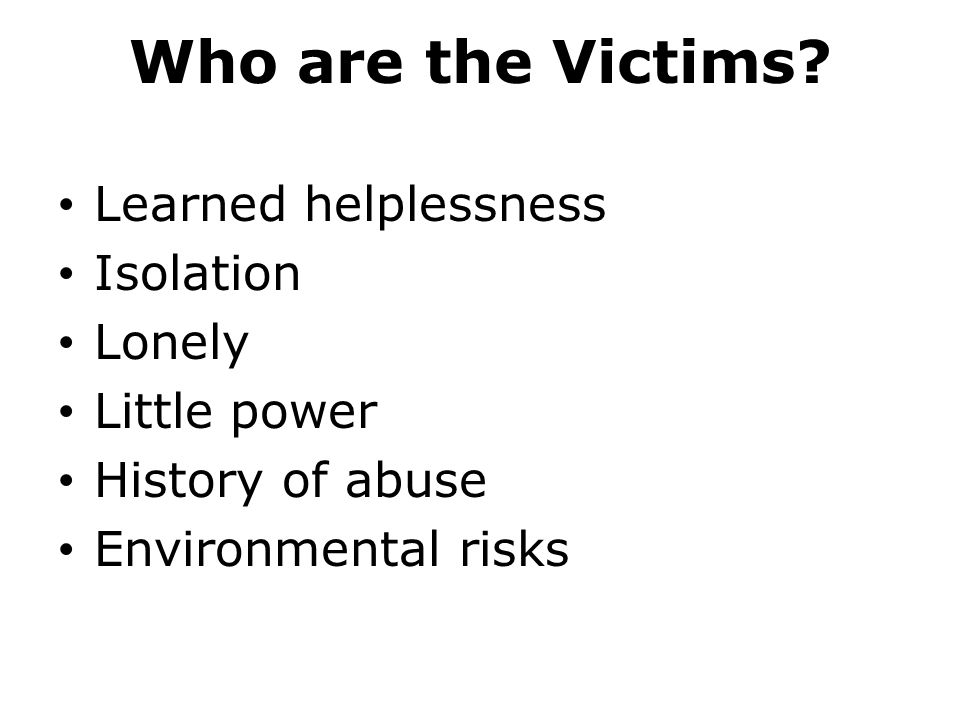The image consists solely of textual content on a plain white background with no borders or additional elements. Centered at the top in bold black text is the heading, "Who are the Victims?" Beneath this heading are six bullet points, each in a smaller, less bold black font, aligned to the left. The bullet points list the following: "Learned Helplessness," "Isolation," "Lonely," "Little Power," "History of Abuse," and "Environmental Risk." Each bullet point starts with a capital letter, and the text appears to be in a sans-serif font, possibly Arial. This layout suggests it's part of a presentation, likely addressing issues related to abused women or children.